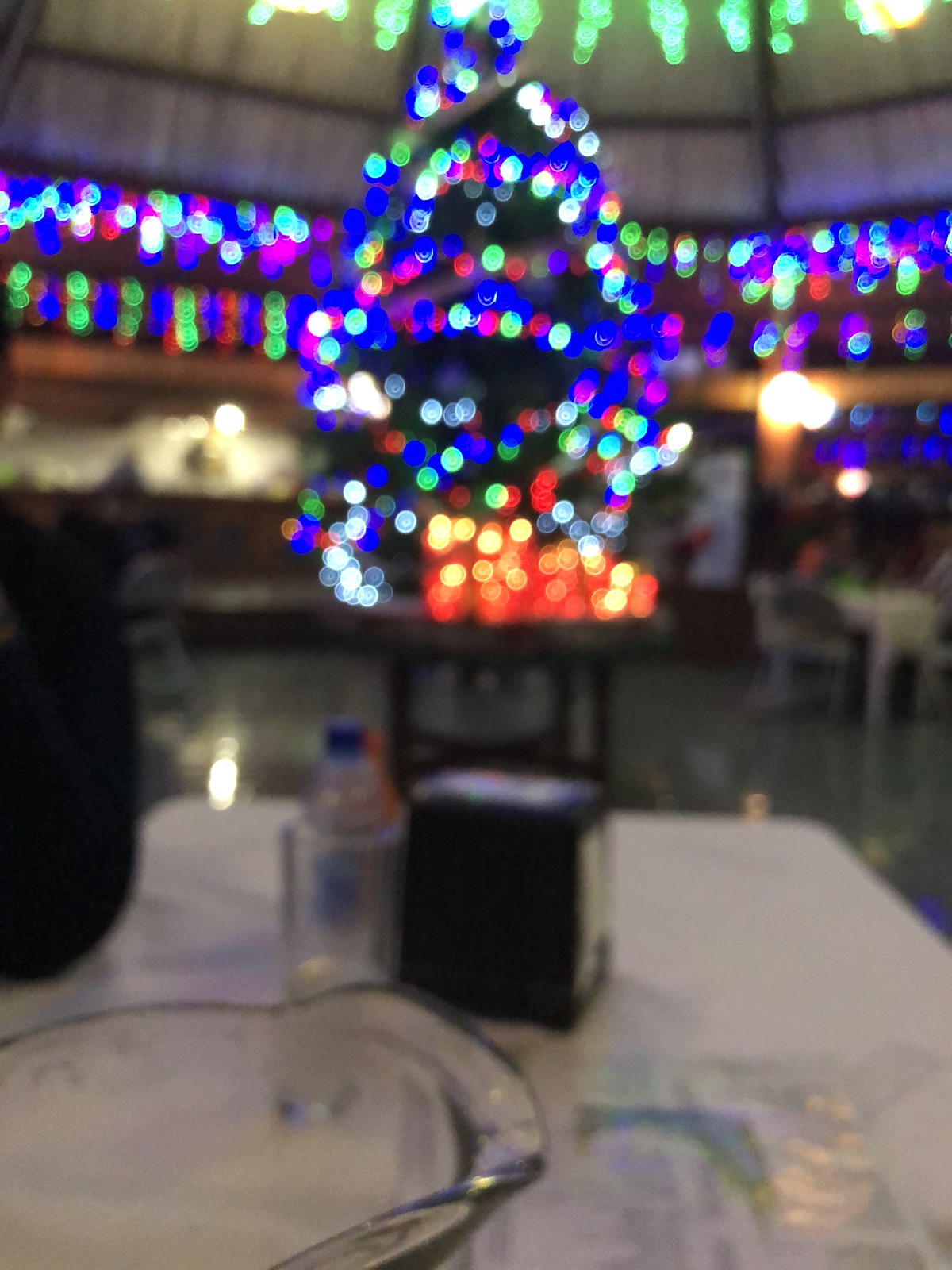This photograph appears to be taken indoors, featuring a somewhat blurry scene. In the foreground, there is a table draped with a white tablecloth. On this table, a glass dish is prominently placed, alongside a clear bottle with a blue lid, possibly a water bottle. Additionally, a black square object, likely a napkin holder, can also be seen. In the background, there is another brown table, which seems to have orange candles or some glowing objects on it. Further in the distance, a multitude of lights create a layered effect, with a predominance of blue lights interspersed with a touch of red.